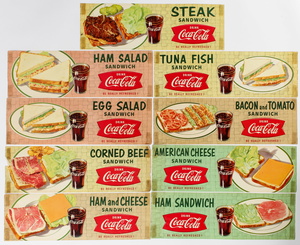This vintage print advertisement features a collection of nine classic Coca-Cola branded signs, each promoting a different type of sandwich alongside a refreshing glass of Coca-Cola. Arranged in a layout of two columns with the ninth sign prominently centered at the top, these signs exude a distinctly retro charm. The topmost sign advertises a Steak Sandwich with a detailed image of a steak sandwich, complete with pickles and lettuce, beside the iconic red and white Coca-Cola logo. Below it, in succession, are ads for a Ham Salad Sandwich, Tuna Fish Sandwich, Egg Salad Sandwich, Bacon and Tomato Sandwich, Corned Beef Sandwich, American Cheese Sandwich, Ham Sandwich, and Ham and Cheese Sandwich. Each vividly colored sign – featuring backgrounds in faded tones of pink, tan, yellow, and green – highlights the respective sandwich plated on a white dish, paired with a tall glass of Coca-Cola. The meticulous imagery includes open-faced sandwiches showcasing ingredients like lettuce, tomatoes, cheese, and ham. This nostalgic collection not only captures the vintage aesthetic of yesteryear but also underscores Coca-Cola’s timeless appeal as a classic accompaniment to a variety of sandwiches.